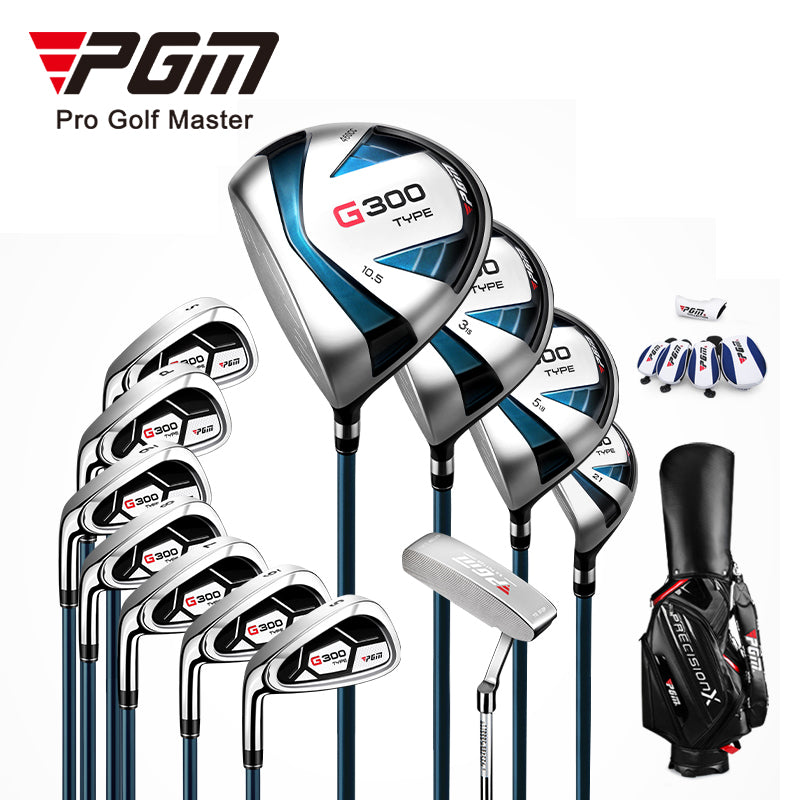This image showcases a comprehensive set of PGM Pro Golf Master golf clubs, perfect for any avid golfer. The set includes four driving clubs and several wedge clubs, all artfully displayed. Highlighted prominently is a putter among the assortment. In the upper right-hand corner, there are stylish blue and white leather covers designed for the drivers. Completing the set is a sleek black golf bag, located in the lower right-hand portion of the image, featuring a shoulder strap and emblazoned with "Precision X" in distinctive writing. The top left corner of the image proudly displays the PGM Pro Golf Master branding, aligning with the array of clubs and accessories that illustrate the quality and variety this collection offers.